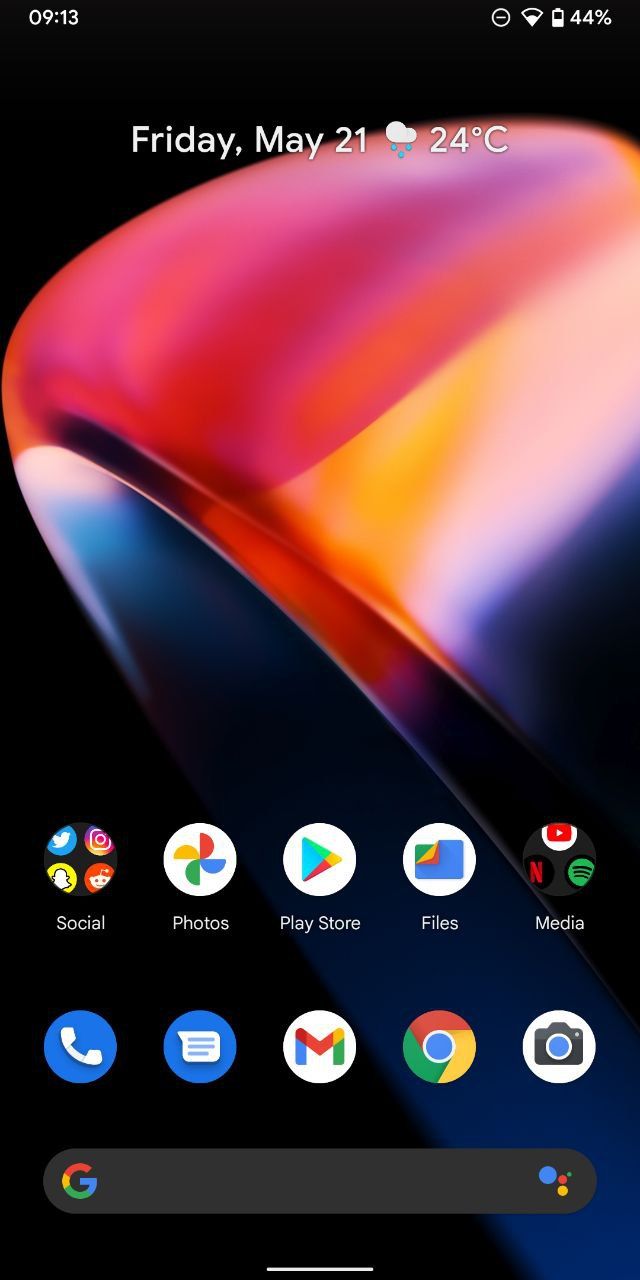The image showcases an Android phone with a distinctive and visually captivating background. The wallpaper features a computer-generated graphic depicting an extreme close-up of a ring at an oblique angle, set against a black background. The ring appears to have a red stone, though it is unclear if the red hue comes from the stone itself or from reflected light. Surrounding the red stone is an abstract, rainbow-like pattern that transitions from red to yellow, white, blue, and violet.

At the top of the screen, the device shows it's 9:13 AM with the Do Not Disturb mode enabled, a weak Wi-Fi signal, and a 44% battery life. The status bar also indicates that it is Friday, May 21, and the weather forecast predicts rain with a temperature of 24°C.

The phone's home screen is notably sparse and minimalist. At the bottom sits the standard Google search bar, an integral feature unless overridden by a third-party launcher. Just above it, there's a non-scrolling dock of frequently used apps, which includes Phone, Messages, Gmail, Chrome, and Camera.

Moving upwards, a single row of additional icons is displayed. The first icon is a folder labeled "Social," containing Twitter, Instagram, Snapchat, and Reddit. Following this are individual apps: Photos, Play Store, and Files. The last icon in the row is a folder labeled "Media," which houses YouTube, Netflix, and Spotify (identified by its recognizable green icon with three black stripes).

This detailed arrangement encapsulates the user’s preference for functionality and simplicity, giving insight into their prioritized applications and overall aesthetic choice.